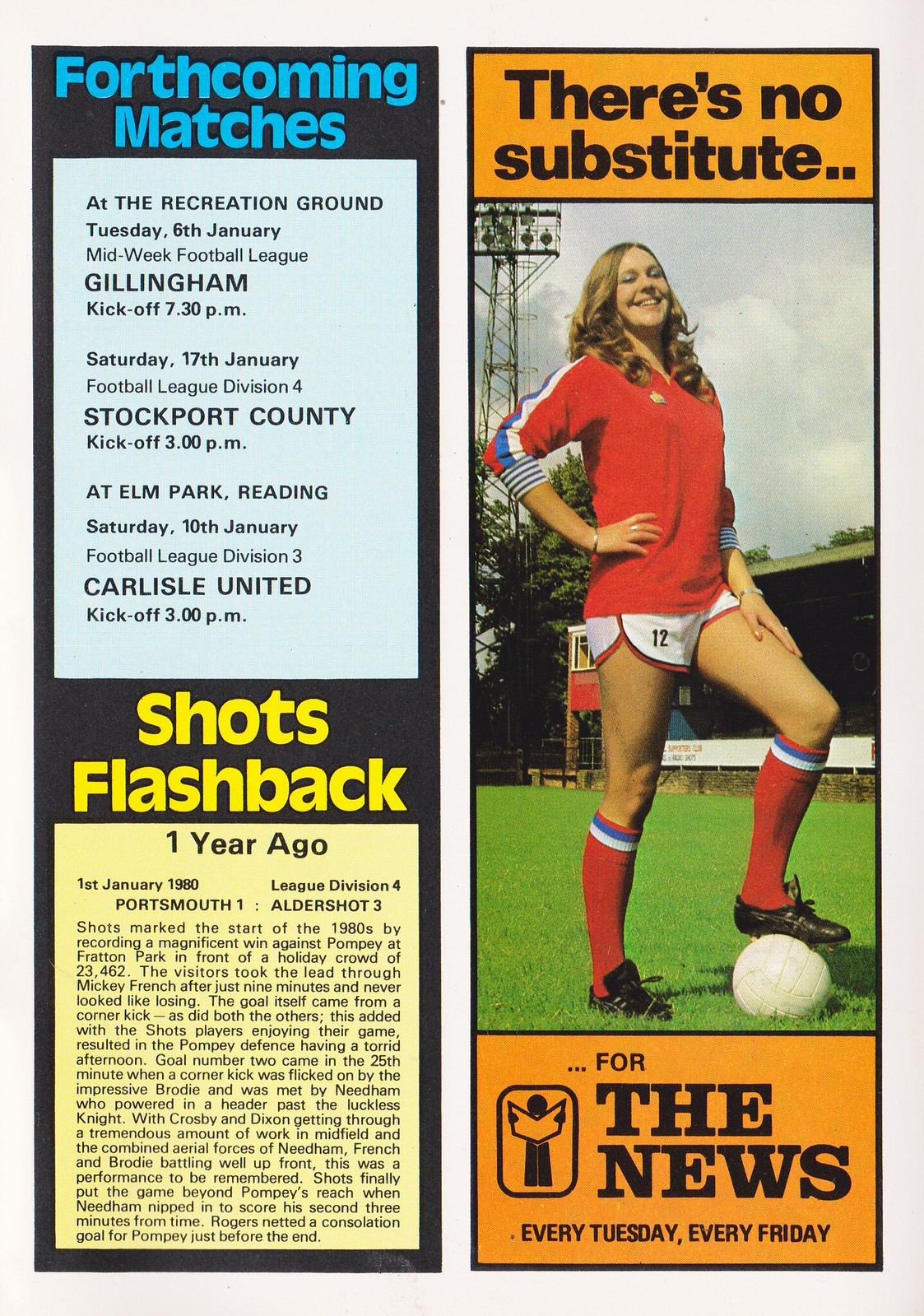The image appears to be an eye-catching vintage poster from what seems to be the 1970s, promoting a women's soccer league, likely in England. Dominating the right side of the poster is a striking visual of a woman standing on a vibrant green soccer field. She is dressed in a distinctive soccer outfit: a red sweater with white, blue, and red stripes, white shorts with the number 12, and knee-high red socks featuring matching stripes at the top. Her long, wavy light brown hair frames her face, and she confidently rests one foot atop a pristine white soccer ball, whilst wearing black shoes. Behind her, a distant tower is visible.

On the left side of the poster, there are two informational segments. The first announces forthcoming matches, listing games at different venues such as Gillingham, Stockport County, Elm Park Reading, and Carlisle United, with specific kickoff times. The second section is titled "Shot flashbacks" and provides a detailed recount of notable games from a year ago, including a match where Outer Shots triumphed over Portsmouth with a score of 3-1.

The header of the poster boldly states "There's no substitute for the news every Tuesday, every Friday," indicating that this advertisement works in tandem with a bi-weekly sports news publication, which chronicles match schedules and past glories. The entire composition employs a palette of red, blue, white, yellow, and black, evoking a vibrant and nostalgic atmosphere.